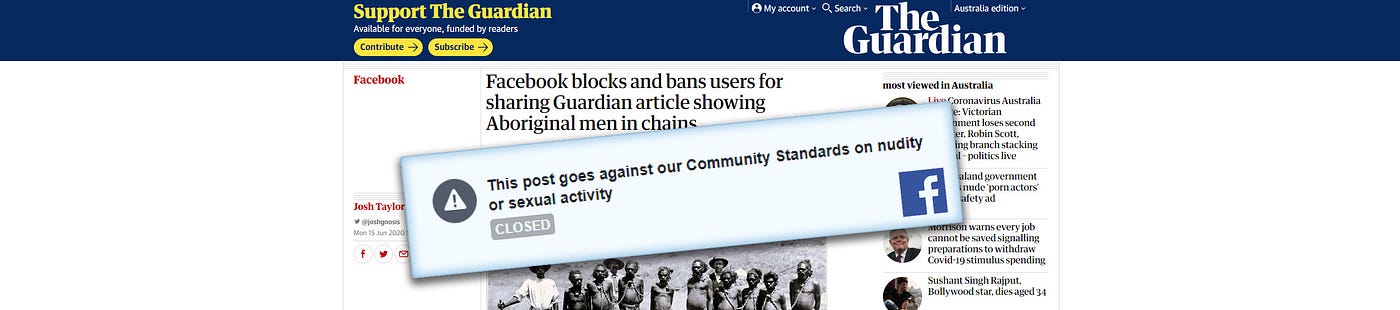The image is a horizontally rectangular screen capture from the upper section of a website. At the very top, there is a narrow, horizontal dark blue banner. Within this banner, in yellow text slightly left of center, is the message "Support the Guardian." Below this message are two buttons labeled "Contribute" and "Subscribe." Just right of center on the same banner is the white text "The Guardian," written in the Guardian's distinctive font.

Beneath this banner, part of an article is visible, though it is obscured by a notification window. The article headline reads, "Facebook blocks and bans users for sharing Guardian articles showing Aboriginal men in chains." This headline is partially covered by the notification window, which appears to be pasted over the article at a slight diagonal angle.

The notification window itself is also horizontally rectangular. To the left, it features a warning triangle icon with an exclamation point inside. The text within the notification states, "This post goes against our community standards on nudity or sexual activity," indicating a restriction or ban by Facebook. At the bottom right corner of this notification window, the Facebook logo is present.